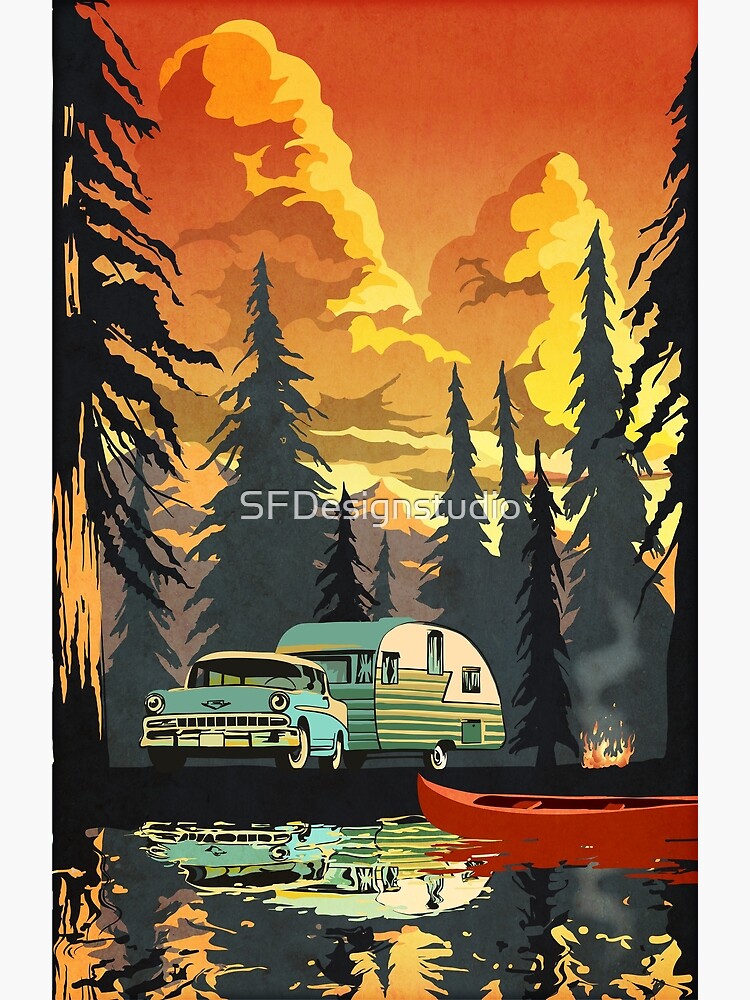This artwork, likely an advertisement for the SF Design Studio, captures a vintage and colorful outdoor scene reminiscent of San Francisco's artistic vibe. Centered around a classic 1950s baby blue Cadillac with a rounded, green and white camping trailer attached, the image exudes nostalgia and style. The vehicle and trailer are parked by a serene lake, their reflections beautifully mirrored in the water. A red canoe is also seen floating on the lake, adding to the picturesque setting. Surrounding the main figures are several tall pine trees, both in the foreground and as dark silhouettes in the background, solidifying the forested campsite ambiance. A small campfire with orange, red, and yellow flames and wisps of smoke sits on the right side, while the sky above features a vibrant sunset with stylized fluffy, orange, and yellow clouds. The whole scene is bathed in the warm hues of a setting sun, bringing a soft, enchanting glow to the landscape. At the center of this elaborate setting, the SF Design Studio logo stands out, integrating seamlessly into the emotive and detailed depiction.